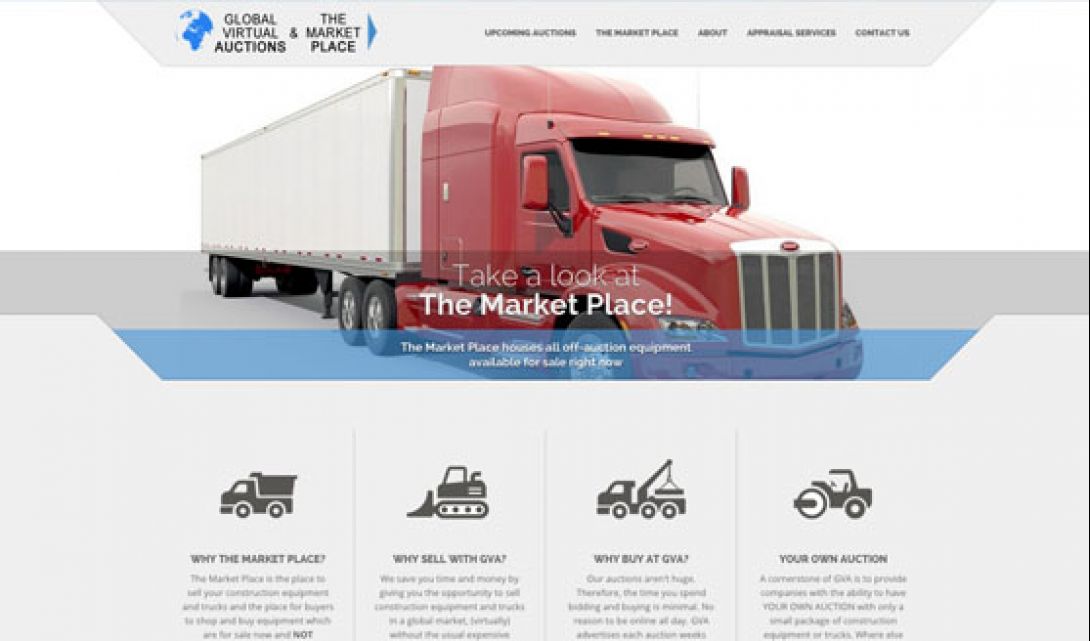A screenshot captures a webpage with a gray header at the top. The header features black and blue elements, including a circular globe icon with blue depictions of various continents. To the right of the globe, black text reads "Global Virtual Icons in the Marketplace." Adjacent to this, a blue arrow points to the right.

The top navigation bar includes tabs labeled "Upcoming Auctions," "The Marketplace," "About," "Appraisal Services," and "Contact Us."

Dominating the page is a striking image of a large red semi-truck viewed from the front, featuring a silver grill. Attached to the truck is a white shipping container with the text "Take a Look at the Marketplace" written in white across a blue banner.

Beneath this are various icons representing different pieces of equipment, including a semi-truck, a bulldozer, a tow truck, and a tractor. Text informs visitors that "The marketplace holds all of auction equipment available for sale right now."